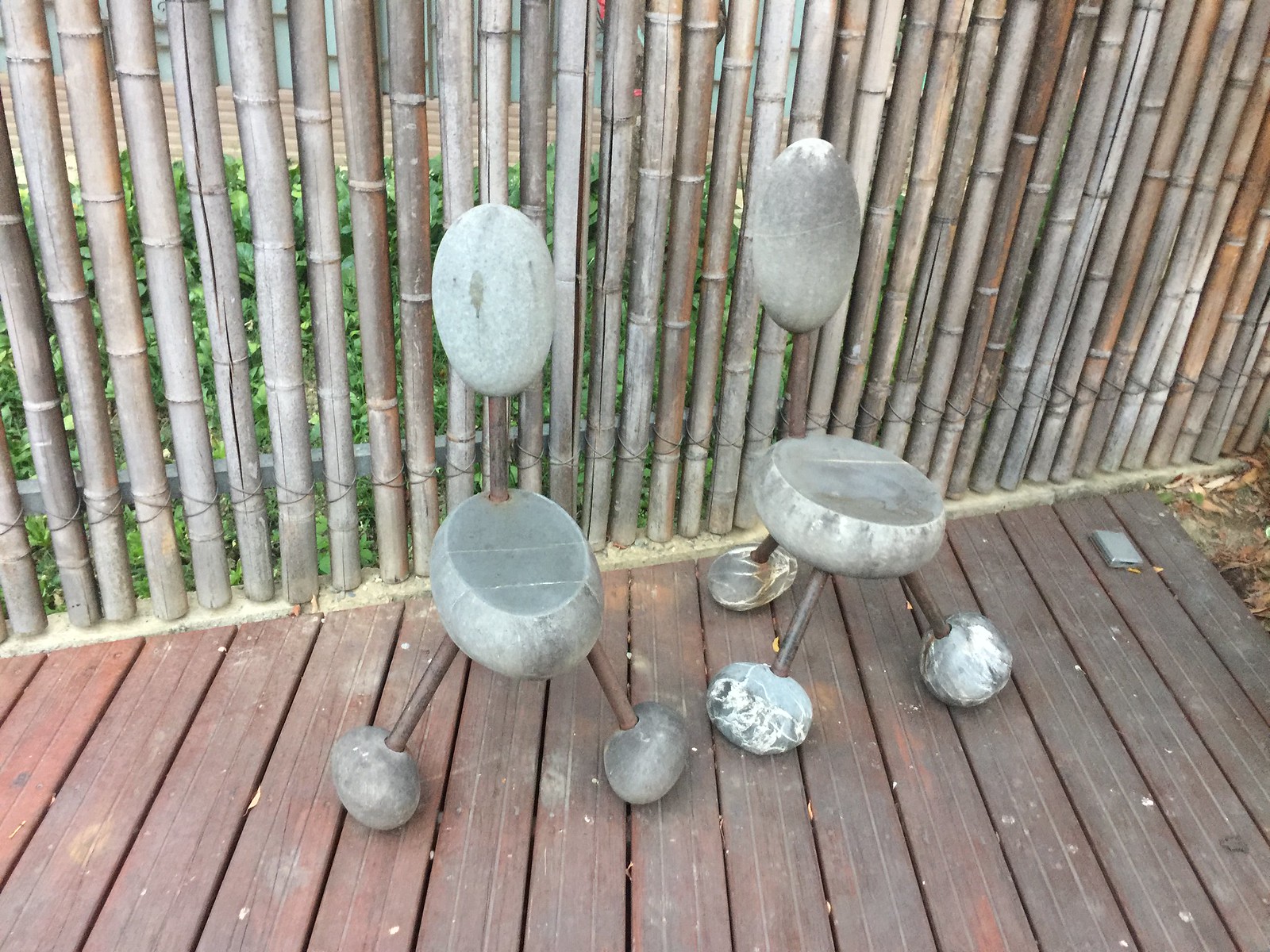On an aged, redwood deck, worn to a mottled reddish-brown and darkened with use, sit two minimalist stone chairs. These unique chairs are constructed of steel tubing and rocks, each featuring three legs formed from rusty steel poles. The backrest of each chair is a large oval rock, drilled and mounted atop one of these poles. The left chair's seat is a large, flat-topped oval rock, while the right chair boasts a nearly perfectly round, lighter-colored stone seat. Each chair’s three steel legs are splayed in a triangular layout, with large rocks attached at the ends serving as feet. The earthy tones and rustic textures of the chairs complement the background, a weathered bamboo fence, rolled out and variegated in shades of white, black, and dark brown. Through the gaps in the bamboo, a garden or yard is faintly visible, hinting at a serene outdoor space beyond.